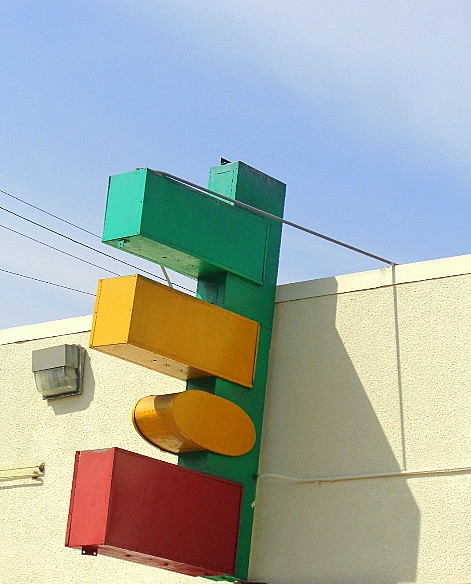The image showcases a side view of a white building with a rough, pebbled exterior. Prominently, a green metal post with variously shaped metal containers attached is being hoisted up or down the building's side using a heavy rope. The surface of the building also features a light fixture and some wires, all painted to match the white exterior. Shadows from the light fixture, the rope, and the object with containers are cast onto the building, adding depth to the scene. The backdrop reveals a clear blue sky with visible cables, possibly electrical or telephone wires, stretching across the left portion of the image.